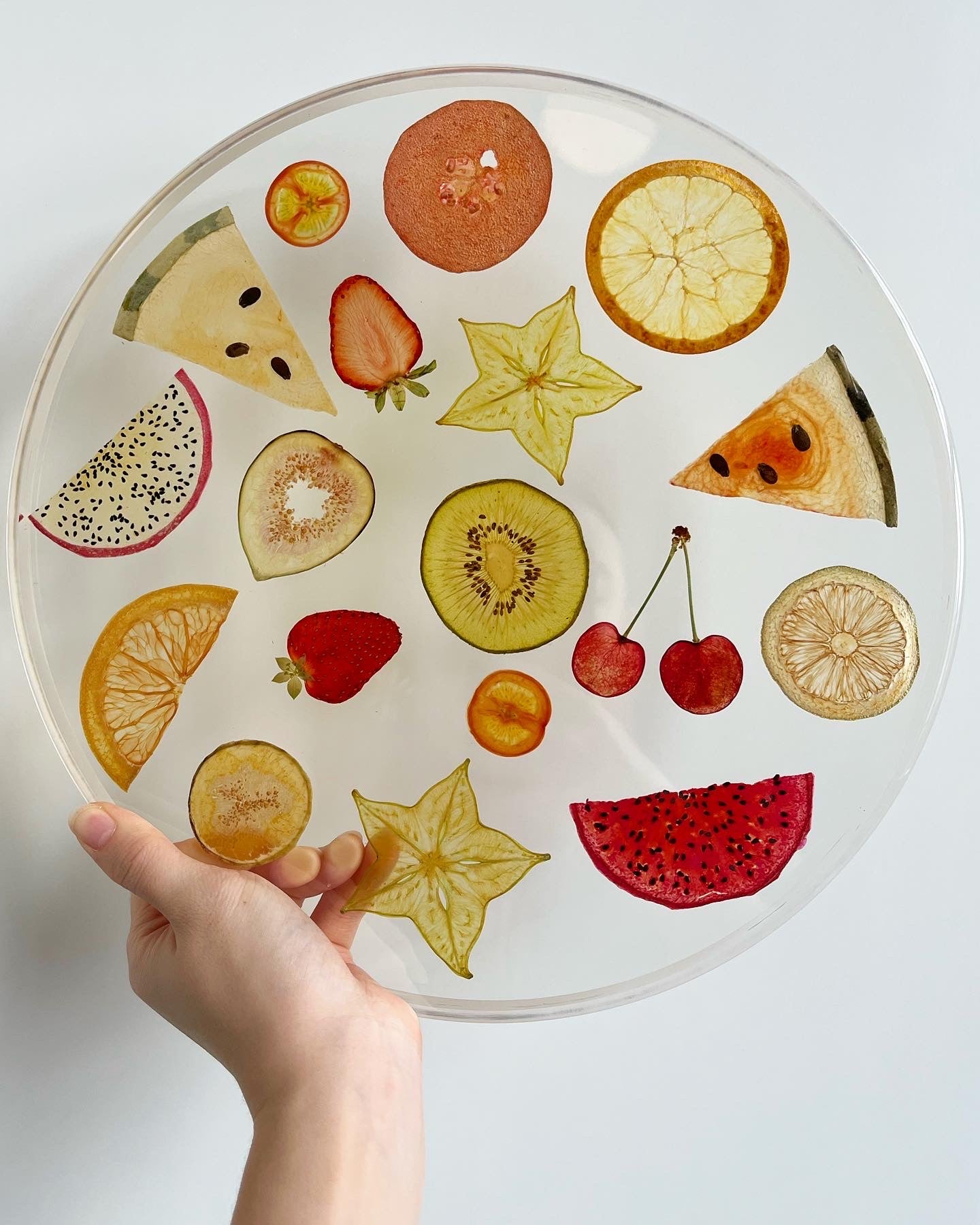In the image, a man's hand and wrist emerge from the bottom left, gripping a round, glass tray with his thumb on top and fingers wrapped underneath. The tray, resembling a microwave plate, is held against a light gray background without any border or text. This glass plate is adorned with colorful, painted images of various foods. At the top, there's a brown cookie, followed by a star-shaped leaf, a sliced strawberry, and a piece of sliced kiwi. To the right, two cherries hang from a shared stem, and above them rests a slice of watermelon. A full strawberry with its leaves is in the lower left, adjacent to a wedge of lemon and another star-shaped leaf. Additional food illustrations include a pomegranate, an orange, and a white half-circle outlined in red with black dots, possibly representing a different fruit or food item. The vibrant colors of the painted foods stand out vividly, contrasting against the light-colored background.